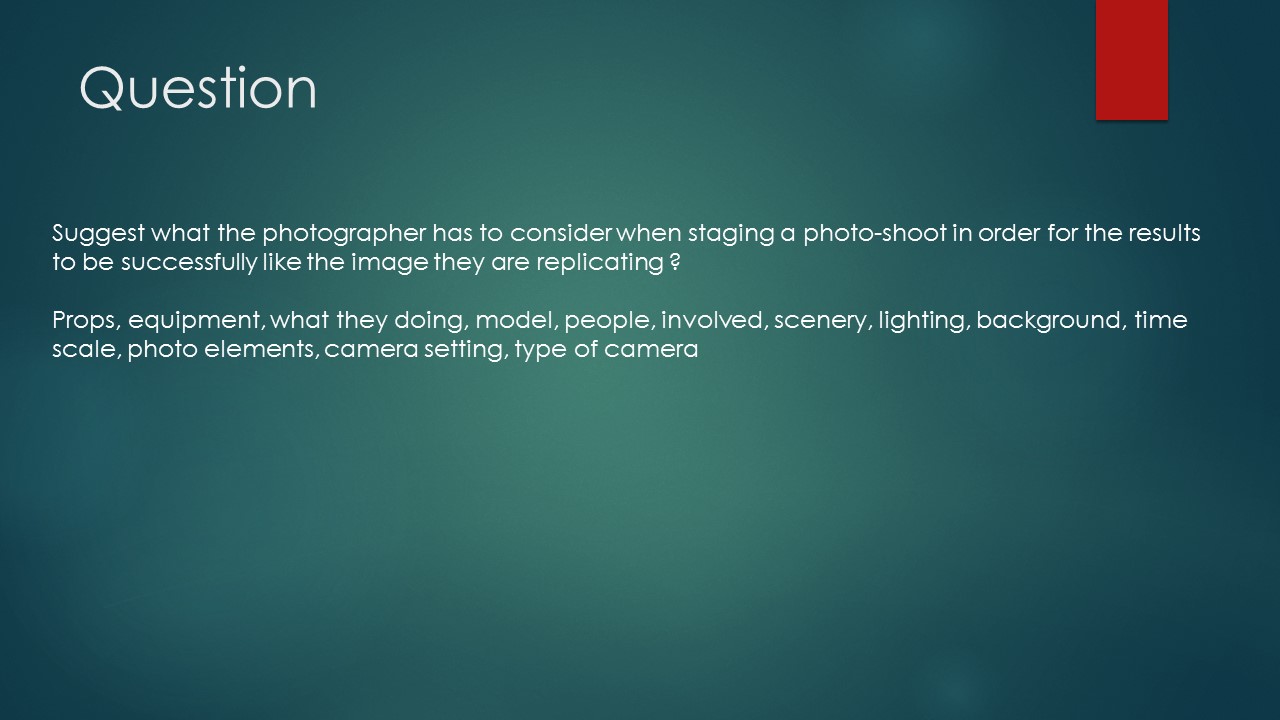The image resembles a PowerPoint presentation slide with a rectangular shape and a greenish background that fades to a lighter green in the center. The title, "Question," is prominently displayed in white text in the top left corner. Below the title, in smaller white text, is the instruction: "Suggest what the photographer has to consider when staging a photo shoot in order for the results to be successful like the image they are replicating," followed by a detailed list of considerations: props, equipment, activities, models, people involved, scenery, lighting, background, time, scale, photo elements, camera settings, and type of camera. This text is organized into two paragraphs. Additionally, the top right corner of the slide features a red horizontal bar about one inch in length, adding a visual contrast to the green background.